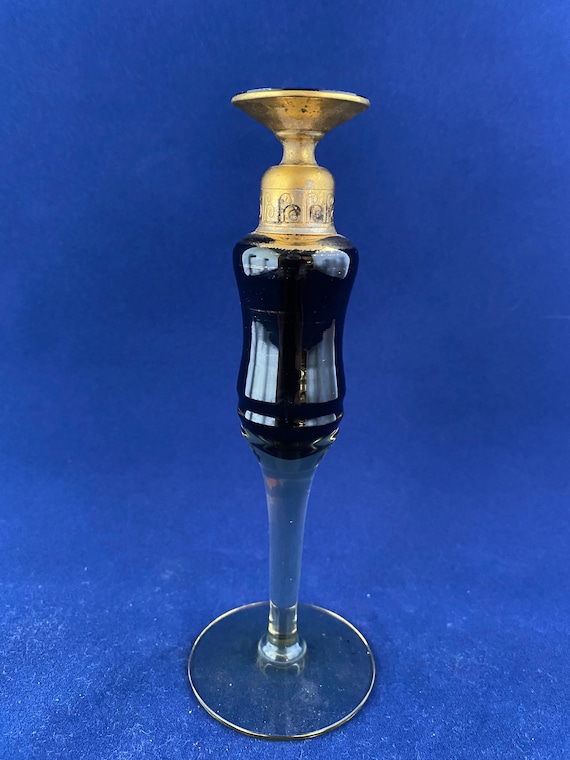The image depicts a unique decorative object featuring elements that make it appear somewhat like a hybrid between a candle holder, an oil lamp, or a piece of decorative glassware. Its structure starts with a base resembling a wine glass, made of clear glass and rimmed with gold. This base supports a black central section, creating a contrasting core. Extending upwards from this section is an ornate gold piece with intricate filigree details, contributing to its decorative appeal. The topmost part is also gold and is complemented by a thin black rim, suggesting it might serve as a holder for something, possibly a candle. The entire object is set against a rich, dark blue textured background, making its colors—blue, gold, and black—stand out prominently.